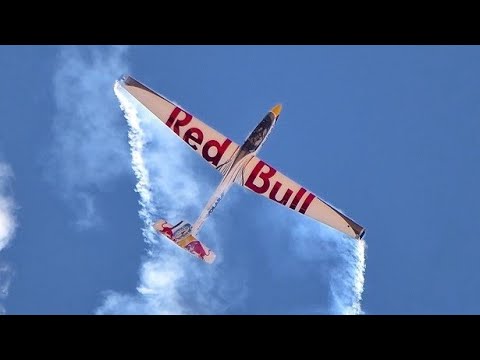This image captures a white, unpowered glider taken from below as it soars through a clear blue sky. The plane is prominently branded with red "Red Bull" lettering across its long wings, with "Red" on one wing and "Bull" on the other. The glider, likely a stunt plane, features notable red accents and a picturesque trail of smoke emanating from canisters at the tips of each wing. Its tail showcases a combination of white, red, and goldish colors, while the nose is highlighted in a yellow or gold hue. The cockpit area appears darker, providing a striking contrast against the glider’s body. The image is bordered by black strips on the top and bottom, resembling a screenshot taken from a video player. Contrails and wispy clouds frame the dynamic scene, enhancing the visual impact of the glider performing under a vibrant, azure sky.